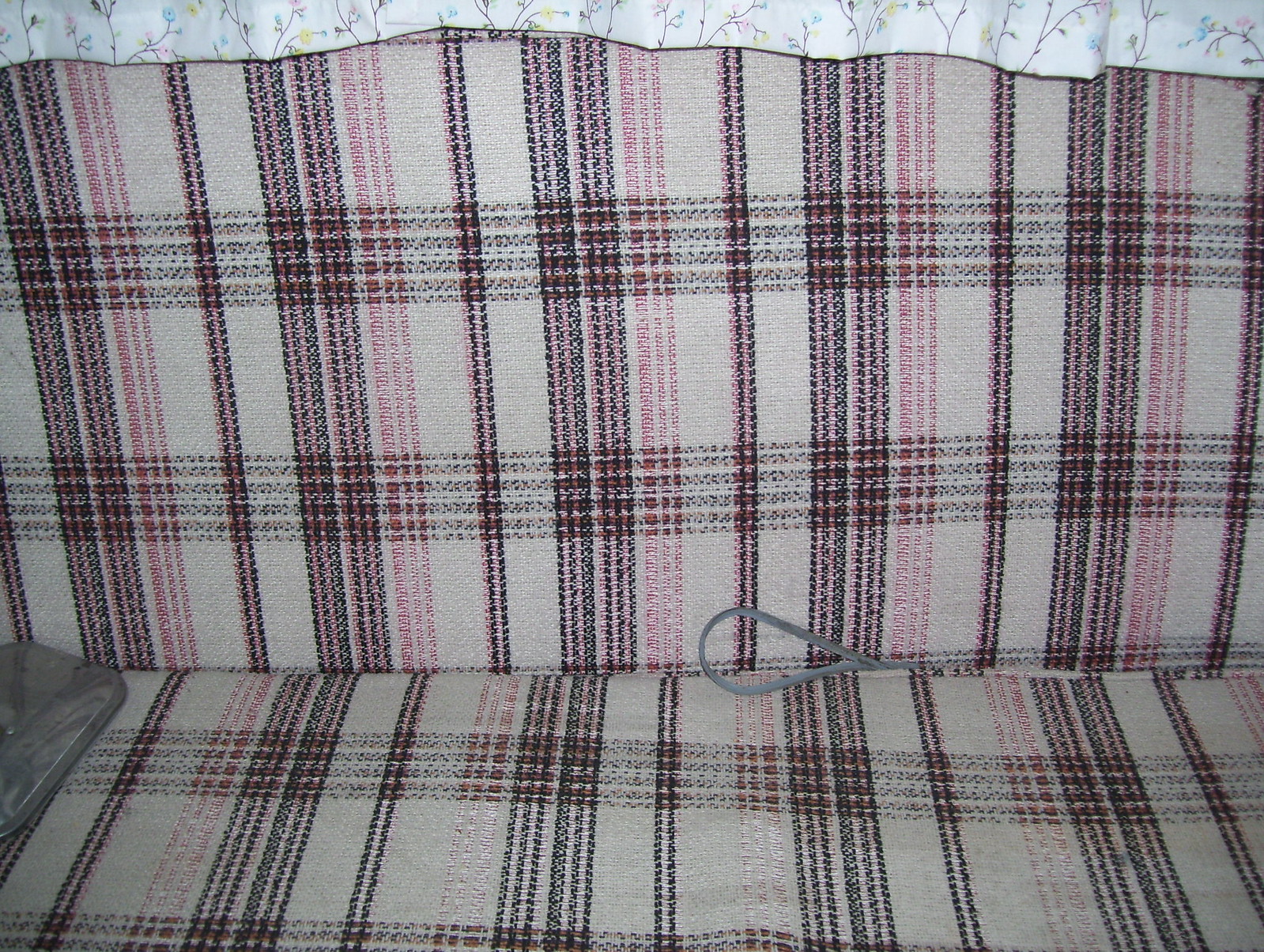The photograph showcases a long sofa or loveseat that spans the entire frame, with visible backrest and seat sections, but no armrests. The sofa is upholstered in a distinct plaid pattern consisting of pink and light brown criss-crossed with white stripes, creating a visually striking design. Draped over the top of the backrest is a white curtain or blanket adorned with a floral pattern of little branches accented by pink, blue, and yellow flowers. On the left side of the seat, there is a gray, flat object that appears to have a zipper around it, potentially a plastic bag. Nestled between the seat cushion and the backrest, a blue loop, likely belonging to a purse or similar item, is partially visible. This blend of colors and textures creates a captivating and detailed composition.